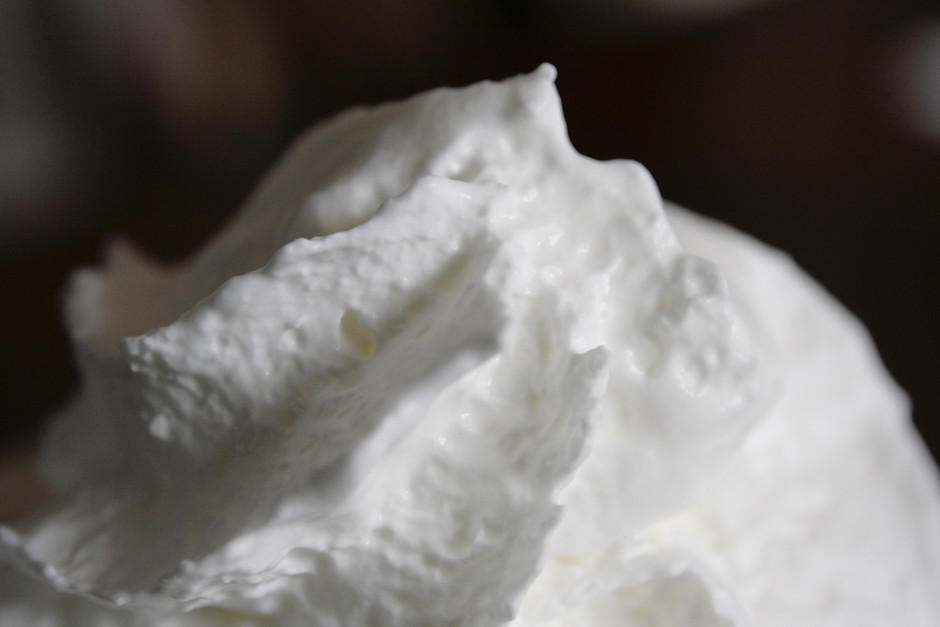This image captures an extreme close-up of a freshly made dollop of whipped cream, likely scooped directly from a spoon. The whipped cream appears fluffy, light, and airy, with visible tiny air pockets scattered throughout, giving it a cloud-like texture. The top of the dollop features a distinctive point and ruffled ripples, particularly towards the left side. The right side has a blurred, smooth roundness, suggesting the motion of it being spooned onto a plate. The background is a blurred mix of colors, predominantly a brownish hue, with some white and green tones and a white half-circle in the right corner, enhancing the soft, ethereal feel of the whipped cream against the contrasting backdrop.